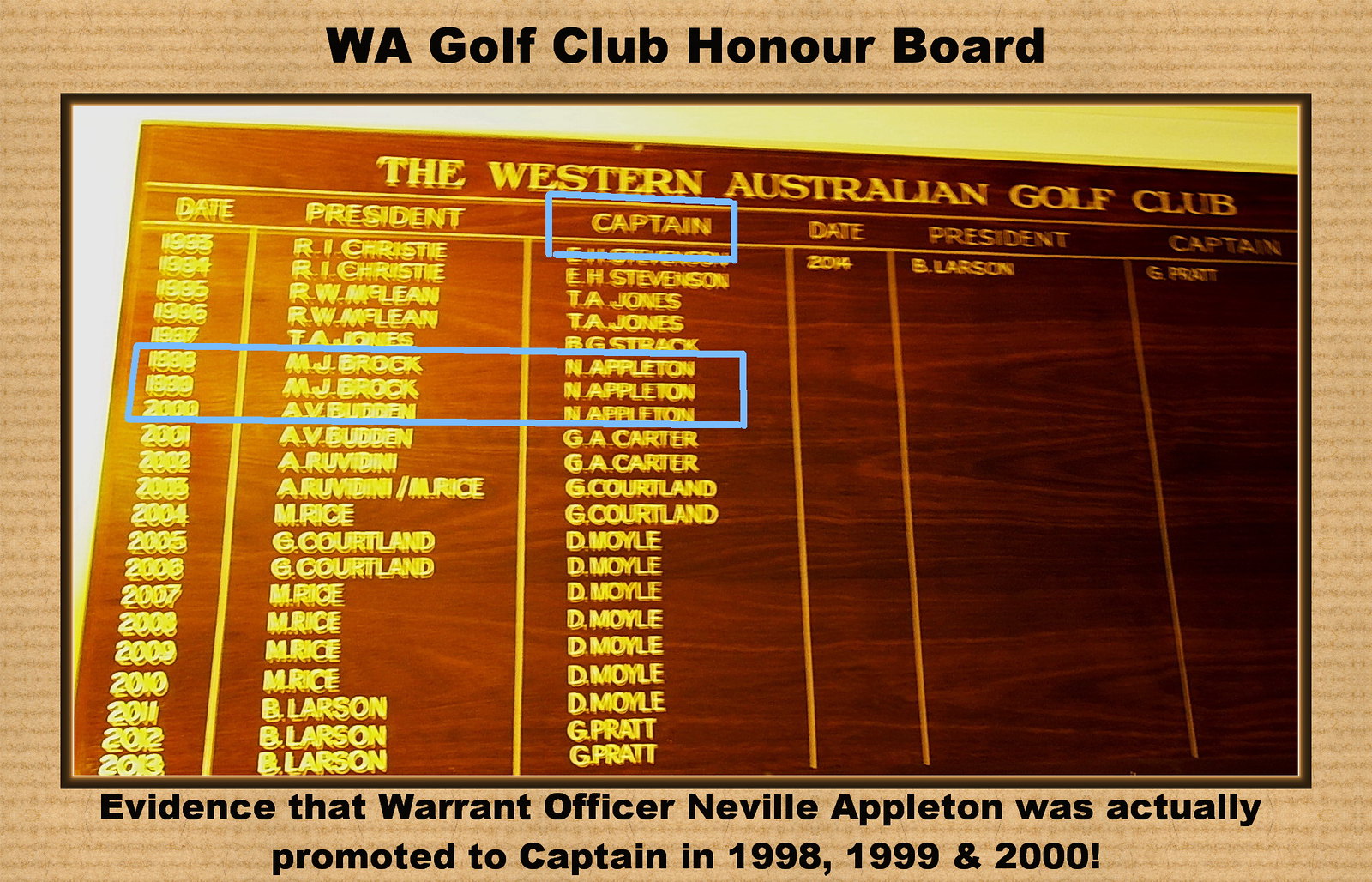The image depicts a detailed honor board on display at the Western Australian (WA) Golf Club. The board, crafted from redwood with a grainy texture, features the club's name "The Western Australian Golf Club" prominently at the top in elegant gold lettering. Below this title, the board is organized into columns labeled "Date," "President," and "Captain," all in gold text. The listed names of presidents and captains are in yellow lettering, arranged vertically under their respective headings. A notable detail on the board is the recognition of Warrant Officer Neville Appleton, who is recorded as having been promoted to captain in the years 1998, 1999, and 2000. The dates and names are encased in a bordered format, adding an official and structured look to the board. The surrounding wall is painted yellow, complementing the brown and gold tones of the honor board, and creating a distinctive, visually appealing display.